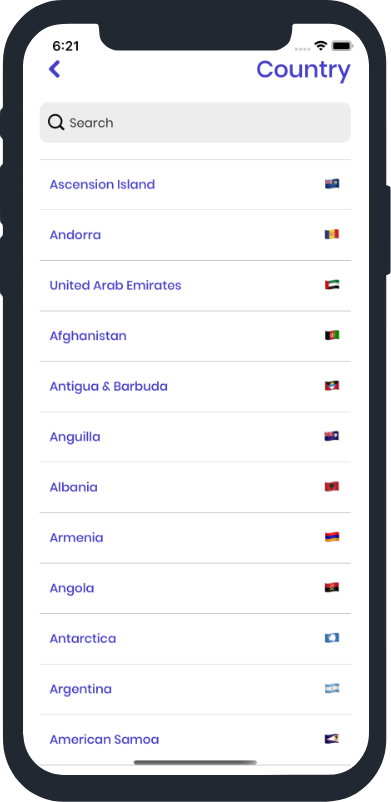The image showcases a detailed illustration of a cell phone screen, featuring a dark gray bezel surrounding the display. The bezel includes three buttons, with two small ones positioned near the top left and one significantly longer button situated on the right. A small black tab extends from the bezel at the top center, slightly overlapping the screen.

The screen itself has a white background. In the top left corner, the time is displayed as '6:21' in black text. On the top right, there are four light gray dots aligned horizontally, followed by a black Wi-Fi icon and a fully black battery icon beneath it. Below this, 'Country' is written in blue text on the right side of the screen, complemented by a blue left-pointing arrow on the left side.

Below this header, there is a light gray rectangular search box with rounded corners, featuring a dark gray magnifying glass icon on the left and the word 'Search' with a capital 'S' next to it. Underneath the search box, a list of countries is presented, with each location name in blue text. The list includes Ascension Island, Andorra, United Arab Emirates, Afghanistan, Antigua and Barbuda, Anguilla, Albania, Armenia, Angola, Antarctica, Argentina, and American Samoa. Each country name is accompanied by a corresponding flag to its right, and the names are separated by thin horizontal light gray lines.

At the bottom of the screen, a medium gray horizontal line is centered, adding a finishing touch to the image.